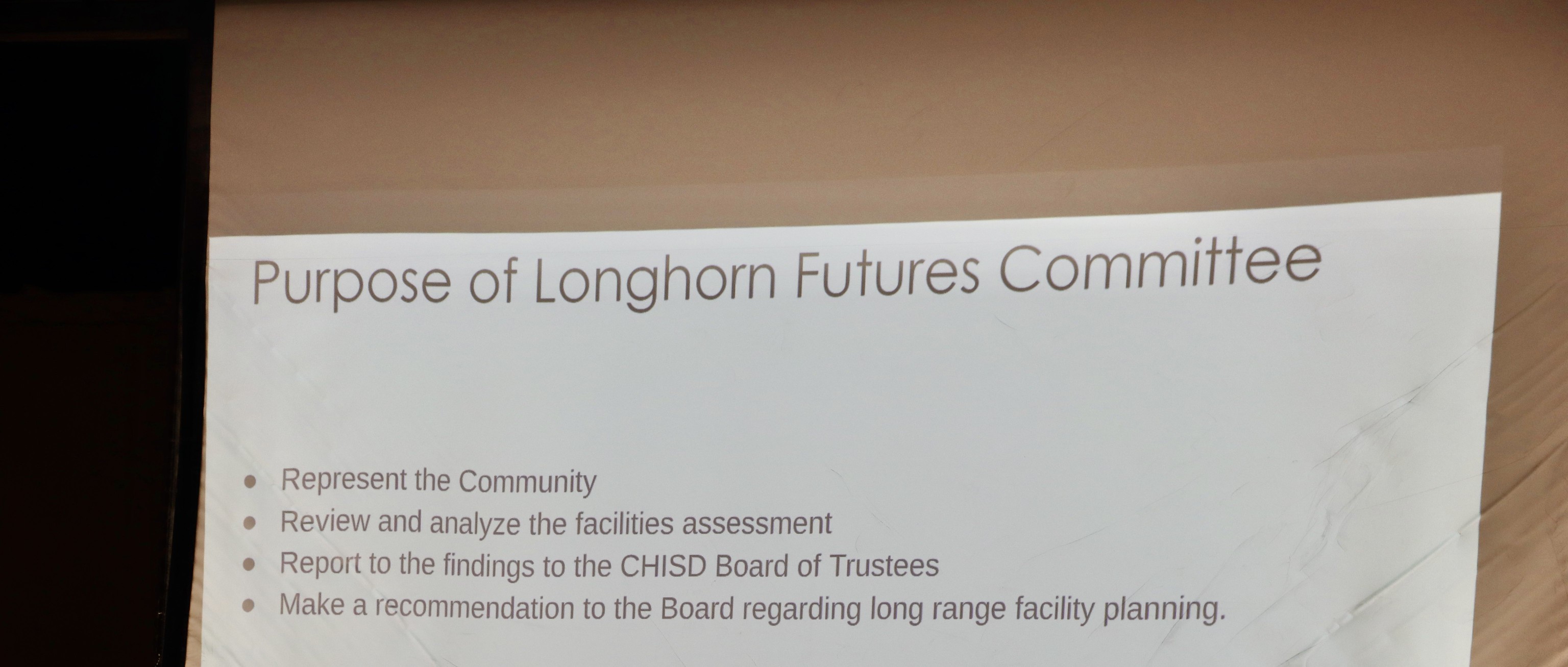This photograph captures a projection screen at an event, likely a presentation, with a black left side and a tan background, possibly a wall or tabletop. The projected white image with black text bears the headline "Purpose of Longhorn Futures Committee." Beneath this title, there are four bulleted points: "Represent the Community," "Review and Analyze the Facilities Assessment," "Report Findings to the CHISD Board of Trustees," and "Make a Recommendation to the Board Regarding Long-Range Facility Planning." The image appears slightly cropped at the bottom, focusing on the presented information's key aspects.